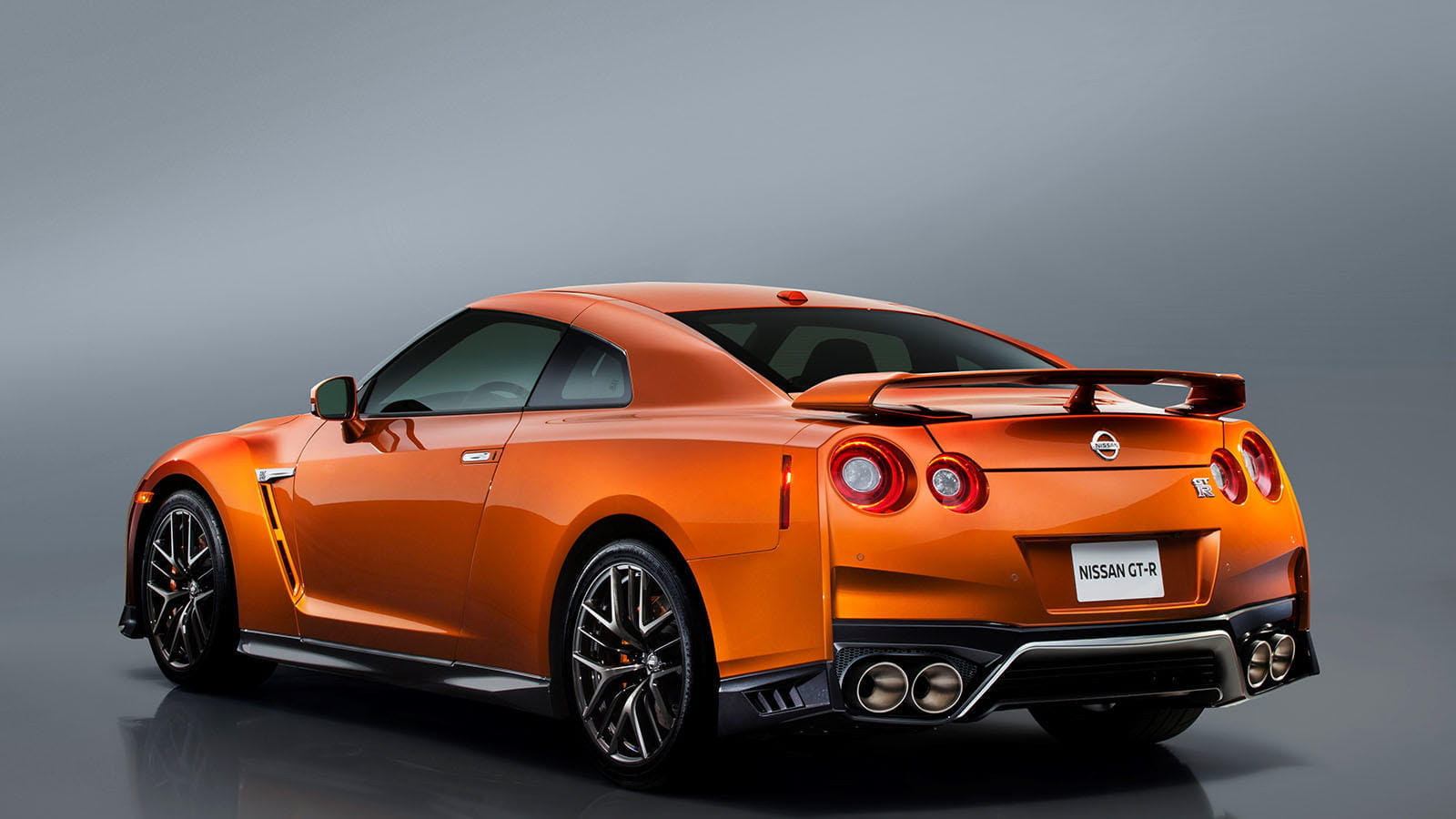The image showcases a vibrant, sporty, metallic orange Nissan GT-R positioned against a light gray background. The car, facing slightly away, exposes its sleek rear, which features a prominent spoiler and a white license plate marked “Nissan GT-R.” The vehicle’s compact two-door design is accentuated by its tinted windows and intricately designed black and silver rims, paired with low-profile tires. Four brake lights and quad exhaust pipes, two on each side, mark its high-performance character. The highly polished and visually striking car appears to be part of a modern promotional image, possibly a digital render or a stock photo for advertising.